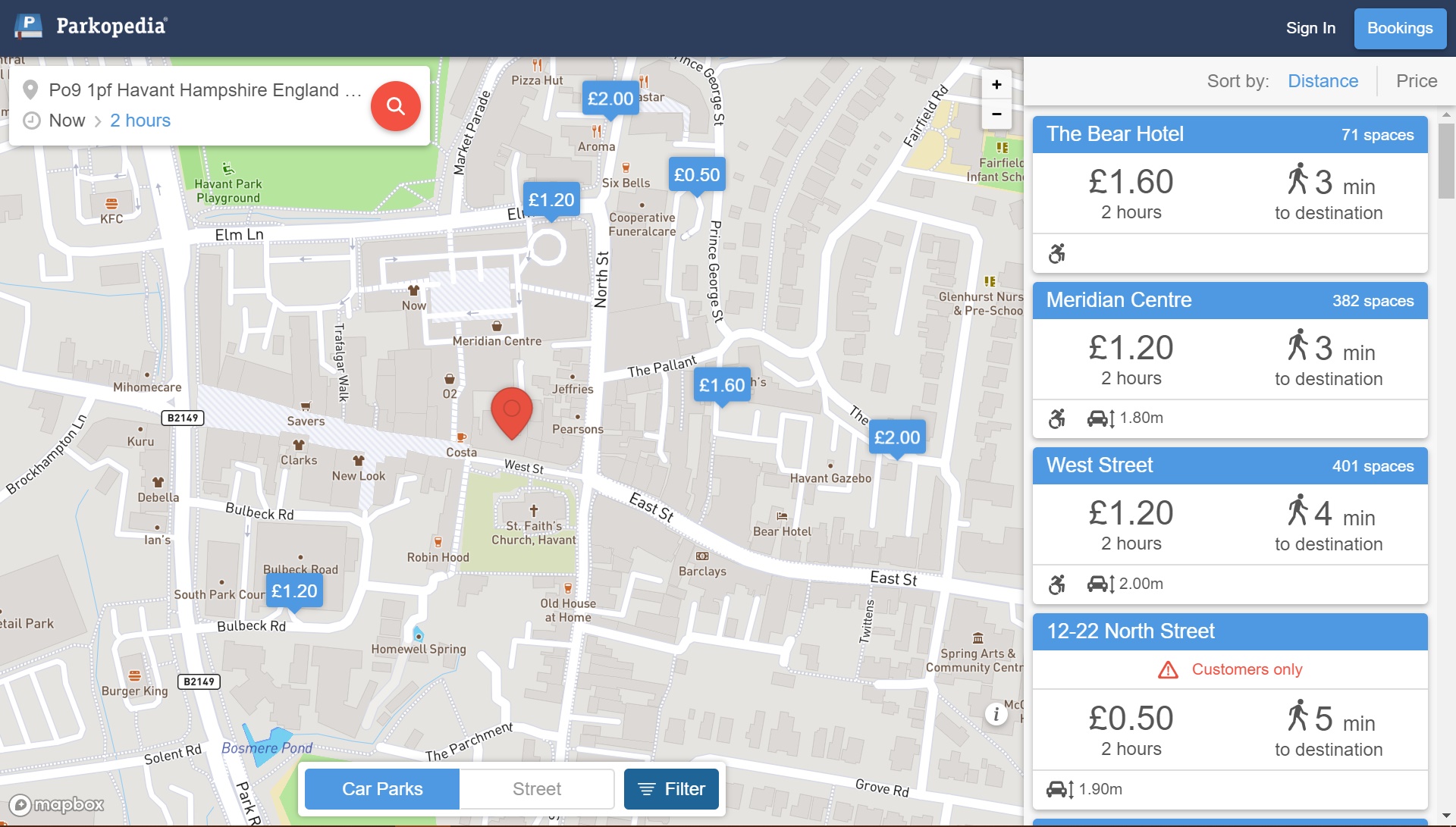This image is a screenshot of the Parkopedia website interface. In the upper left corner, the logo is visible, featuring a book with a letter 'P' on it. The upper right corner displays options to 'Sign In' and 'Bookings'. On the left side of the interface, there is a map with an address in the upper left section, marked with various blue rectangles indicating different parking locations and their prices.

On the right side of the screenshot, a detailed chart lists several parking options and their respective details. The first entry is 'The Bear Hotel', with a fee of 1.60 euros for 2 hours and a distance of 3 minutes to the destination. The second option is 'Meridian Center', costing 1.20 euros for 2 hours, also 3 minutes away. The third listing is 'West Street', priced at 1.20 euros for 2 hours and 4 minutes from the destination. The final entry shows '12-22 North Street', available for customers only, charging 0.50 euros for 2 hours and situated 5 minutes away from the destination.